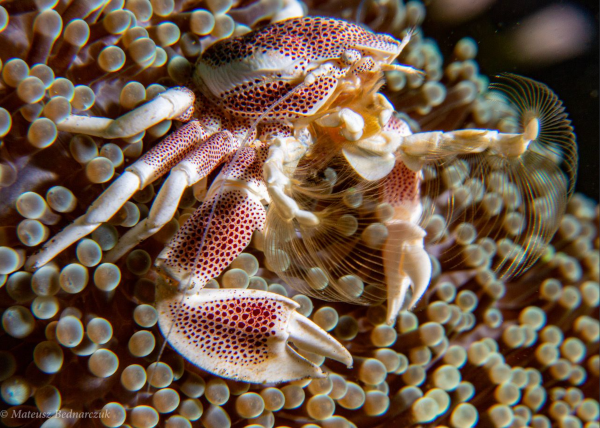The photograph captures a close-up view of a porcelain crab, centrally positioned, amidst a marine backdrop. The crab exhibits a striking appearance with a predominantly ivory-colored, delicate shell, accentuated by dark pink maroon speckles and a subtle blush of light red beneath these spots. Its claws, featuring this distinct spotted pattern, are located towards the bottom of the image, while some legs extend to the left, showing similar coloration and detail.

Surrounding the crab are numerous tiny spherical or tubular structures that resemble beige and translucent globules or possibly crab eggs, contributing to the textured and intricate sea floor background. The image features lighting, likely sourced from the left, casting a gentle glow on the crab, enhancing its porcelain-like appearance. The upper right corner remains blurred and darker, contrasting with the more detailed and illuminated sections. Notably, the image includes a copyright symbol on the lower left corner, attributed to Mateusz Bednarczyk. The photograph vividly depicts a serene marine life scene, focusing on the refined details of the crab and its aquatic surroundings.